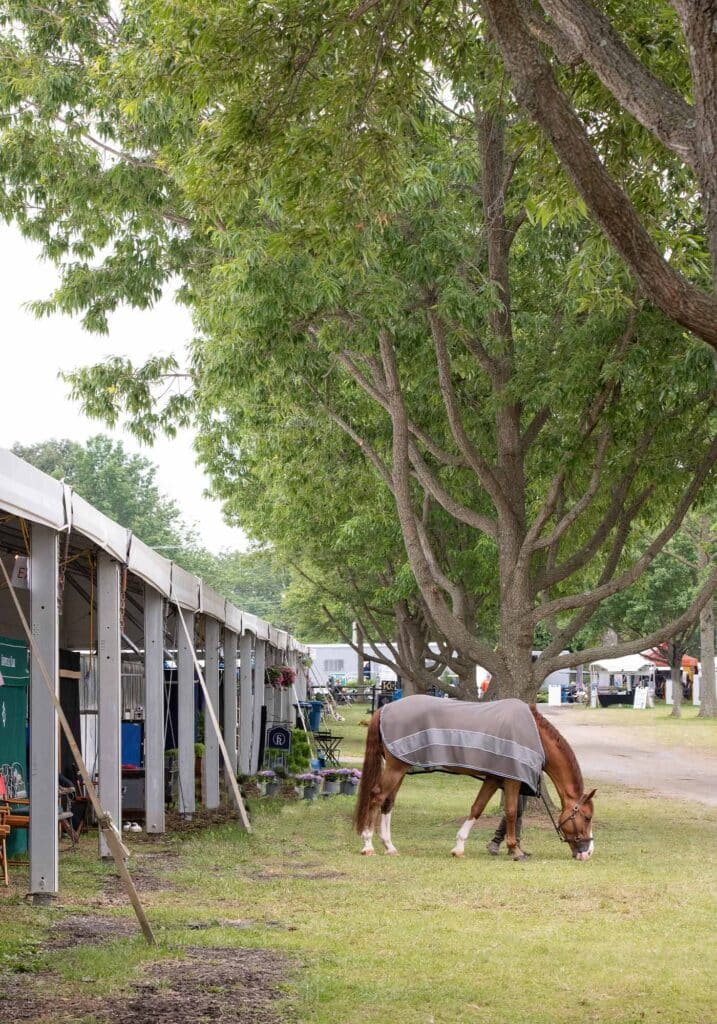In this outdoor photograph, a brown horse, wearing a gray weather jacket, is chewing on short, almost yellow-brown grass interspersed with patches of dirt. The horse stands prominently in the center, against a backdrop of a large oak tree with green leaves and curved branches, positioned to the right. To the left of the horse, there is a short gray building resembling a stable with open slats, appearing temporary and tent-like with a canvas roof supported by metal beams. On the right side, a narrow pathway is visible. The scene is under a gray, steely sky that suggests impending rain or a dreary day. In the background, across the field of grass, there are mobile homes and additional trees, further setting the scene.